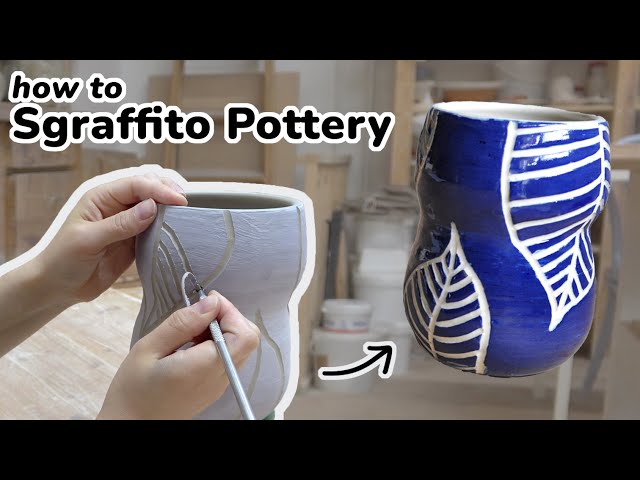In the center of the horizontally rectangular image, framed by thick black borders at the top and bottom, two white hands engage in the intricate process of sgraffito pottery. The hands, outlined in white for emphasis, grasp a metal carving tool with a hooked end, meticulously etching leaf patterns into a grayish, unfinished clay pot. This pot, held steady by one hand from the top edge, contrasts with its finished version indicated by a black arrow pointing upwards to the right. The completed pottery piece showcases a smooth, shiny blue glaze, with etched white leaf designs. The text, "How to Sgraffito Pottery," appears at the top right in prominently outlined black letters. The backdrop, slightly out of focus, suggests a busy art room filled with wooden tables, stands, buckets, and shelves, contributing to the instructional and workshop atmosphere of the scene.